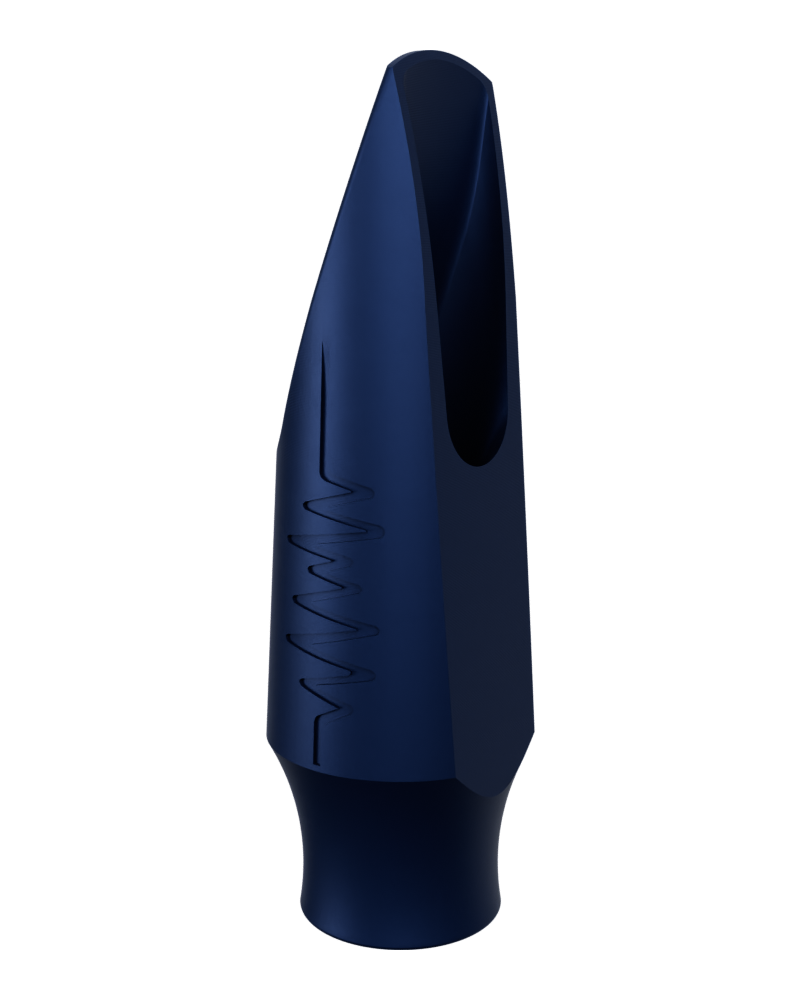The image depicts a black plastic mouthpiece that resembles an attachment for a wind instrument, perhaps akin to a tuba. The mouthpiece stands on its flared base, extending upright into the air, and is characterized by a tapered design leading to a hole at the top where one would blow air into. This air would then travel down into the tube part that connects to the instrument. The mouthpiece features intricately carved lines that start straight before becoming squiggly, resembling sound waves or seismic waves, running along its side. The overall form, with its circular base and rounded front, may also evoke comparisons to a vacuum cleaner hose attachment, notably with an oblong opening on the right-hand side and a wavy pattern on the left, suggesting a multifaceted ergonomic design exposed to air on one side.